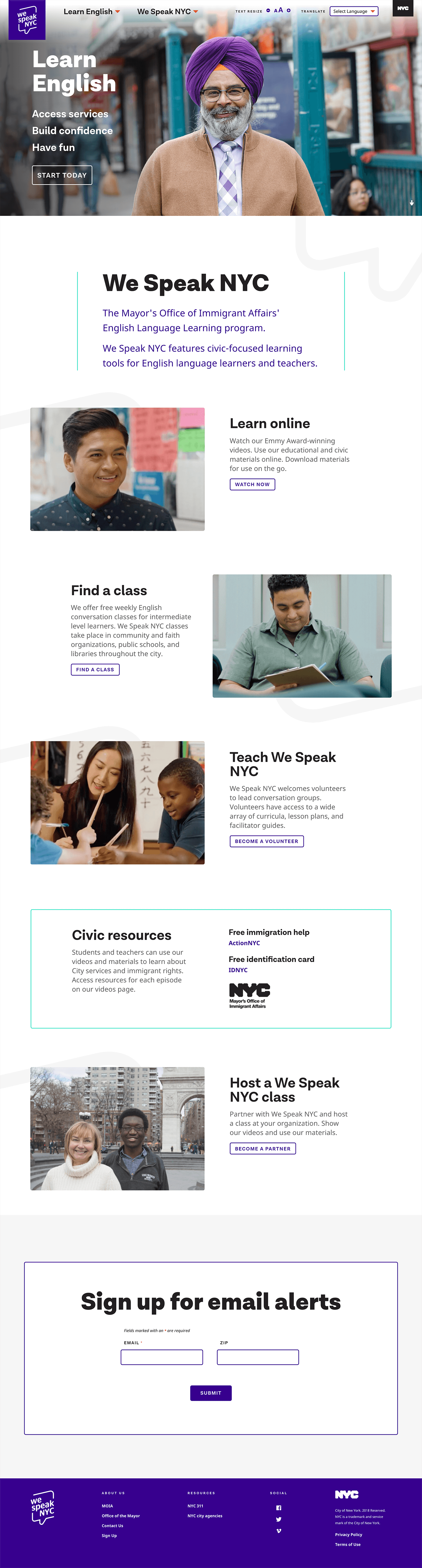This image is a screen capture likely taken from a mobile phone, showcasing a webpage from the "We Speak NYC" website, which supports English language learning and access to civic services. At the top of the page, there is a photograph of a man wearing a purple head scarf, a purple tie, and a tan jacket. Below the image, the text reads "We Speak NYC, the Mayor's Office of Immigration Affairs, English Language Learning Program." The program offers civic-focused learning tools for English language learners and educators.

Underneath, there are several sections: 

1. **Learn Online:** Accompanied by a picture of an Asian man.
2. **Find a Class:** Featuring what appears to be an Arab man engaged in learning.
3. **Teach We Speak NYC:** Next to a photograph of an Asian woman.

Below these sections, there is a blue box titled "Civic Resources," containing additional information. Further down, there's a picture of a black woman and a white woman, alongside the text "Host a We Speak NYC class." A prominent purple button is also visible in this part of the screen capture.